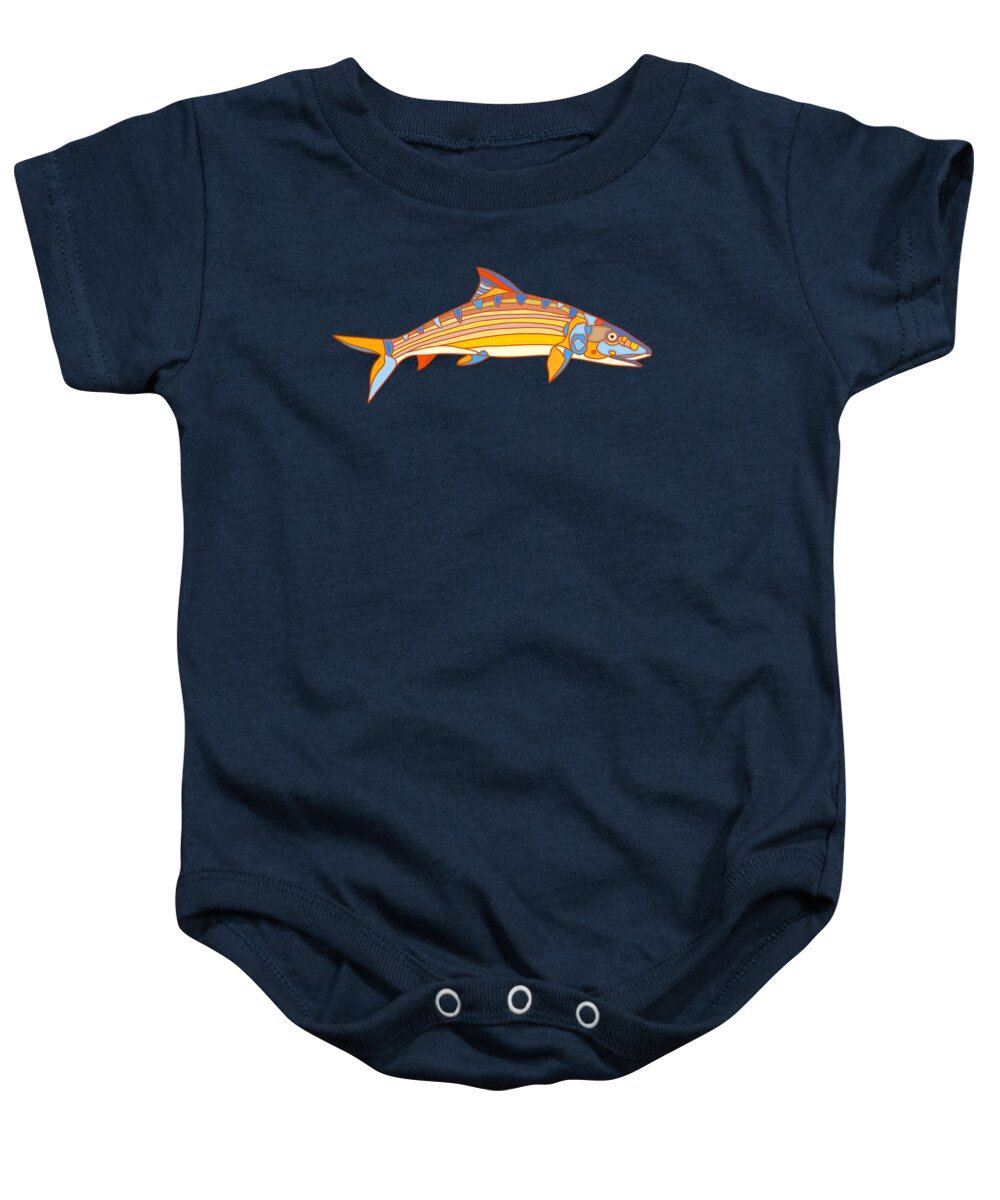The image showcases a short-sleeved, dark blue baby onesie against a pristine white background. The onesie, which appears slightly rumpled, features three press studs at the bottom, each with a white rim, designed to secure the material between the baby's legs. Adorning the chest of the onesie is a striking abstract image of a fish, its head angled toward the right. The fish boasts a vivid palette of colors including orange, yellow and various shades of blue and peach. It has horizontal stripes and blue splotches interspersed across its body, with its top fin and tail exhibiting a mix of orange and blue hues. The fish's mouth is slightly ajar, adding character to the design. This vibrant and playful motif contrasts beautifully with the dark blue fabric of the onesie, making it a charming and eye-catching baby garment.